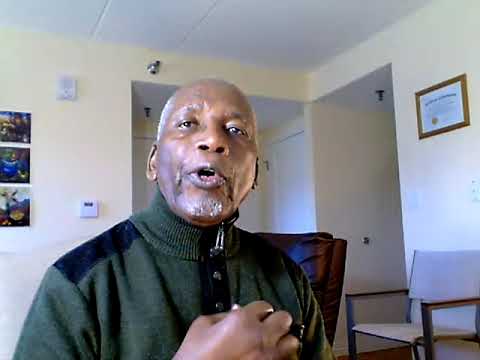The image captures an older Black gentleman, likely in his forties or fifties, seated in a lightly furnished room that resembles an office or den. He is prominently placed slightly off-center to the left, with his face taking up most of the frame. The man is bald with some gray hair around his temples and sports a thin, gray mustache and goatee. He is dressed in a dark green quarter-zip pullover, accented with black patches on the shoulders.

To his left, a dark brown leather chair can be seen partially, while to his right there is a cloth chair set against the tannish-white walls. Above his head hangs a silver fire sprinkler, and on the wall to his far right side, a diploma with a light brown wooden frame is prominently displayed. Behind the chair to his right, the wall seems to extend into a hallway, indicating further space beyond this room. The far left wall holds several blurred pictures or paintings, displaying a mix of colors like blue, green, and white, though they are not clearly visible. The room is softly lit, with a ceiling that's a clean white, completing the setting's subdued and professional ambiance.

Overall, the colors in the image range from the man's brown skin and pink tongue, to his dark green and black clothing, against the neutral tones of the room's furnishings and walls.